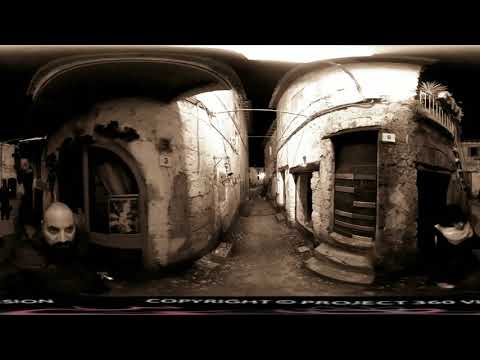The photograph exudes a creepy, eerie vibe, with its predominantly black and white color scheme accentuated by sepia undertones that make it look old-fashioned and outdated. It's a 360-degree image captured inside an abandoned, decaying structure. The stone walls curve around both sides of the scene, creating a hallway-like effect in the middle. On the left side, a large domed window marked with the number 3 is visible, while to the right, a boarded-up door features the number 10. Both of these distinctive buildings flank a long alleyway that vanishes into the distance, where a faint light can be seen. 

In the bottom left corner of the photograph, there is a man dressed in all black, bald, and with dark brown facial hair, seemingly “green screened” into the image. He is holding a camera and his head is slightly turned to the left. Steps lead up to an open door on the right side, and various shades of black, tan, white, and gray enhance the decaying, abandoned feel of the buildings. Additional black bars run vertically at the top and bottom of the image, contributing to its aged appearance.

A light fixture is suspended from the ceiling in the foreground, casting an unusual illumination over the scene. At the very bottom of the photograph, there is a black rectangle with white text that reads "copyright project," adding a mysterious, almost out-of-place element to the unsettling atmosphere.